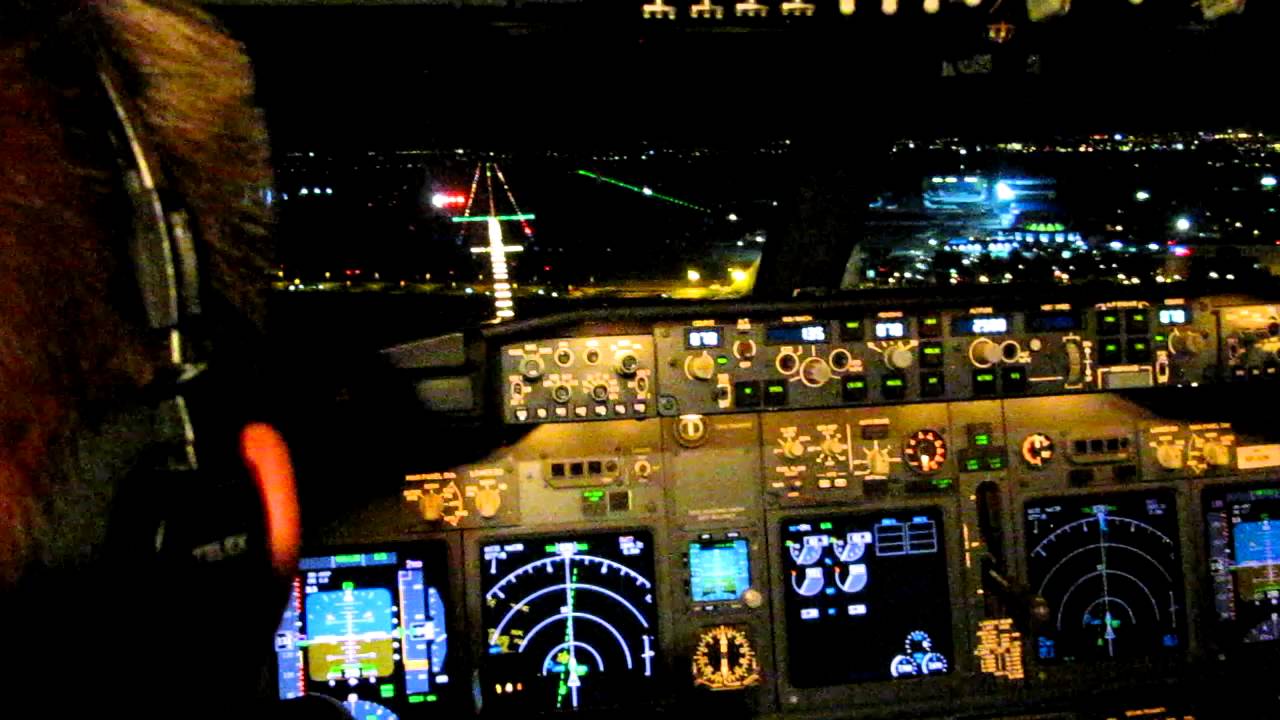This image showcases the interior of a jet airline cockpit at night with a focus on landing. The cockpit is dimly lit, emphasizing the array of illuminated instruments and screens that are casting a soft blue and green glow across the control panels. The control panel, a sizeable rectangular structure predominantly in a gray metallic hue, houses numerous knobs and buttons, each with their specific sections. The screens display various essential data, primarily in black with white and orange numerals and indicators. 

In the left portion of the frame, the back side of the pilot’s head is visible, adorned with short brown hair and wearing a black headset with an orange outer cup. Outside the cockpit window, the runway is clearly visible, lit up against the nighttime backdrop, guiding the plane for its landing. The city or additional sections of the airport stretch into the right side of the frame, adding tiny specks of white and blue lights to the encompassing darkness.